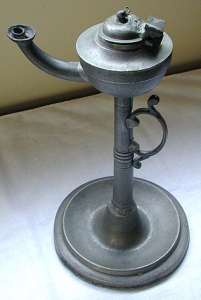This is a close-up photograph of an antique oil lamp that exhibits a tarnished, pewter-like finish, though it may have originally been brass. The lamp stands approximately five to six inches tall and has a rounded, textured base with a distinctive circular layer design. Rising from the center of the base is a lengthy, upward-leading stick that contributes to its vintage appearance. While the glass globe that typically encloses the flame is missing, the lamp still features an ornate handle under the burning mechanism, likely designed to accommodate two fingers. The surface the lamp rests on is white, and there's a tan wall in the background, further highlighting the aged and detailed craftsmanship of this elegant yet weathered piece.